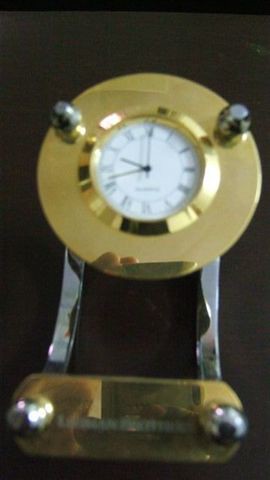The image is a blurry, out-of-focus color photograph of a clock against a black background. The clock appears to be made of a shiny brass, which gives it a golden hue. The clock face is relatively small and features black Roman numerals. It has an hour, minute, and second hand, with the time showing as exactly 9:40. The brass clock is round with a beveled brass circle in the middle. Beneath this central circle, there is a chrome-like piece with legs extending toward the left and right. An oblong brass plaque is mounted horizontally at the bottom of these legs, attached with screws. This plaque bears an engraved name, although it is not readable in the image. The clock may be no taller than a foot, as inferred from a partial reflection of a hand holding the camera in the shiny surface of the clock. Additionally, there are decorative knob-like screws at the top, suggesting this clock could be a special item, perhaps an award or a retirement gift.